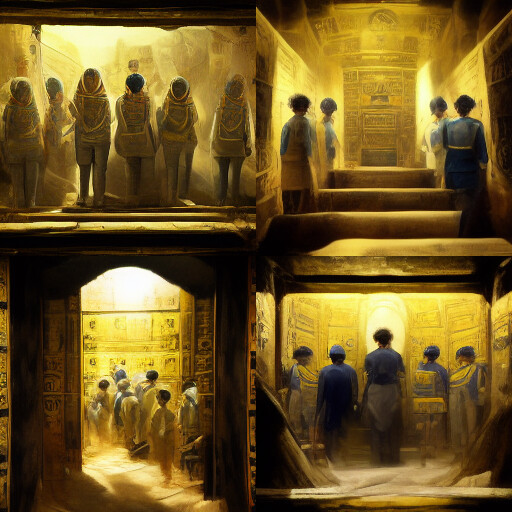The image is divided into four distinct sections, each depicting scenes likely set within a religious or ceremonial structure reminiscent of an Eastern Indian temple, possibly Hindu or Buddhist in nature. 

In the top left corner, six children, dressed in white gauze-like clothing, stand facing the viewer in a room bathed in a golden, well-lit glow. Their solemn expressions and direct gazes create an eerie ambiance.

The top right image portrays four children, positioned two on each side of a stairway that leads to what seems to be an elaborate altar or entryway within the temple. The children appear to be reverently kneeling or standing on the steps.

The bottom left section captures a line of individuals, possibly children, filing through an arched doorway towards a building that emits a mystic, yellow-gold light, emphasizing the sacred or ceremonial nature of the scene.

In the bottom right corner, a group of grown teenagers is depicted, kneeling before a richly ornate altar. The room is adorned with intricate engravings and suffused with a yellow hue, enhancing the sacred atmosphere. One individual is seated in a yellow chair, facing a wall that appears to be decorated with control-like panels, adding a layer of mystery.

Overall, the image vividly conveys a sense of reverence and mysticism within a richly adorned and ceremonially significant environment.